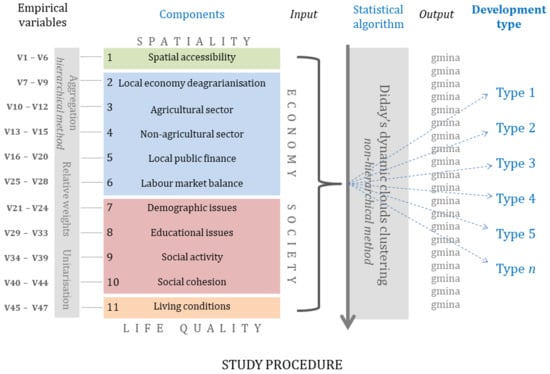The image portrays a detailed scientific diagram titled "Study Procedure" at the bottom in black letters. It features several interconnected sections. The top left section, marked "Empirical Variables," lists numerical variables labeled sequentially from V1 to V47. Adjacent to this, the diagram has a rectangular section titled "Components," followed by a labeled line segment reading "Input." Another rectangular section, noted as "Statistical Algorithm," comes next, leading to an "Output" section. 

The diagram spans across 12 columns and utilizes color-coded bars to distinguish various variables and their categories. These categories include spatial accessibility (green), local economy and deagranization (blue), demographic and educational issues (light red), and living conditions (orange). Additionally, it references concepts such as Dye Day's dynamic clouds clustering and applies a non-hierarchical method to analyze different development types—ranging from type 1 through type 5 and concluding with type N, all written in blue. The contents of the chart primarily feature gray tones, accented with some blue, green, light red, and orange, all set against a clean white backdrop.